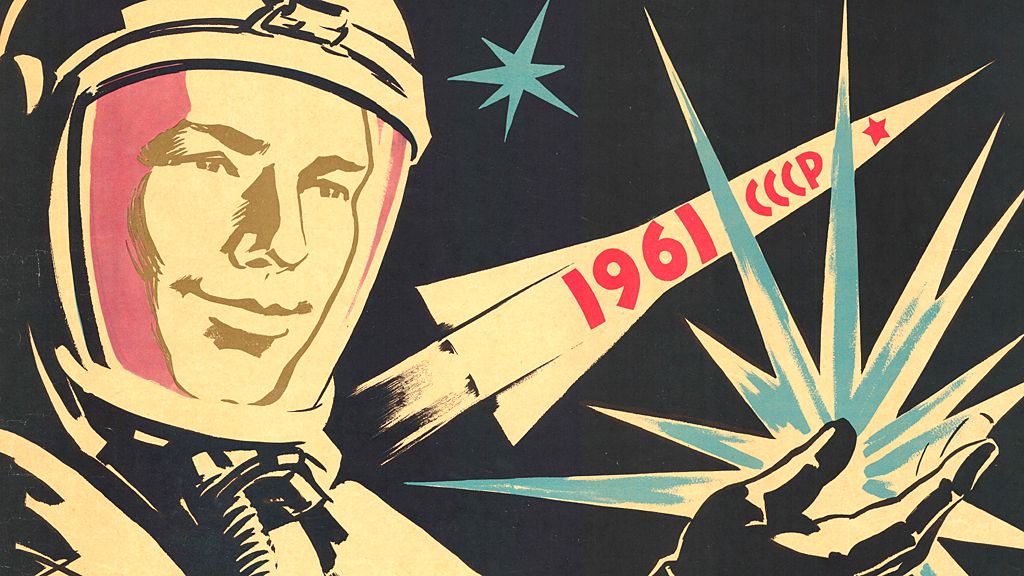The image is an animated, multicolored poster featuring a cartoonized astronaut against a psychedelic backdrop. The astronaut, who doesn't appear to be Chinese, wears a full spacesuit with a helmet featuring breathing tubes and a face shield. He is holding a glowing blue and white star in his hand, which simulates reflection. Above his hand, there is a rocket ship with "1961" and "CCCP" written in red letters, along with a red Communist star symbol. The rocket, emitting steam or flames from its back, appears to be flying upwards beside the astronaut's smiling, upward-facing visage. The scene includes a non-reflective blue star above the rocket and utilizes a color palette of blue, pink, white, black, and tan.